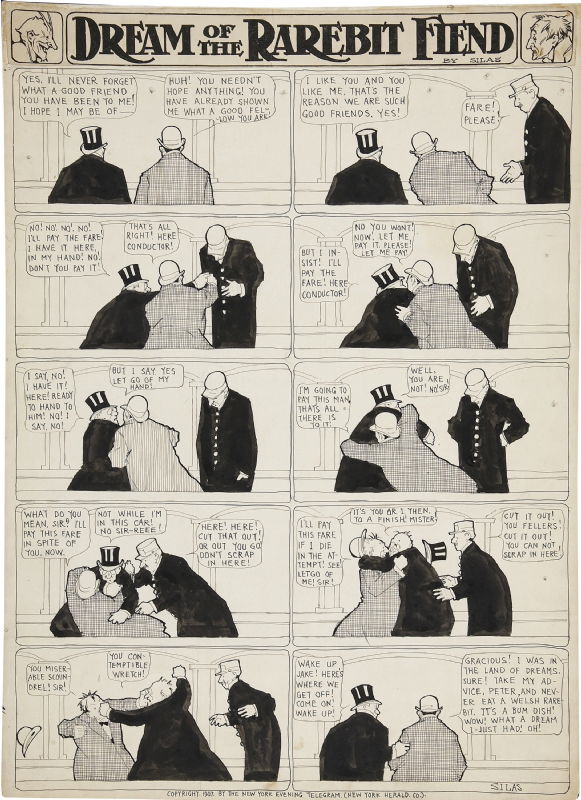The image is a page from the New York Evening Telegram, featuring a vintage comic strip titled "Dream of the Rare Bit Fiend" depicted in black, white, and gray. The comic consists of five panels on each side, narrating the interaction between two men with their backs turned away, seated on a train or bus. One man, wearing a black coat and top hat, begins by saying, "Yes, I'll never forget what a good friend you've been to me. I hope I may be of..." The other, dressed in a plaid or gray coat with a rounded top hat, responds, "Huh, you needn't hope anything. You've already shown me what a good fellow you are." The dialog continues with, "I like you, and you like me. That's the reason we are such good friends, yes?" At this point, a conductor intervenes, asking for the fare. They both offer to pay, leading to an escalating argument and eventually a brawl, with the conductor attempting to break them up. The strip culminates with the two men sitting quietly beside each other once more.